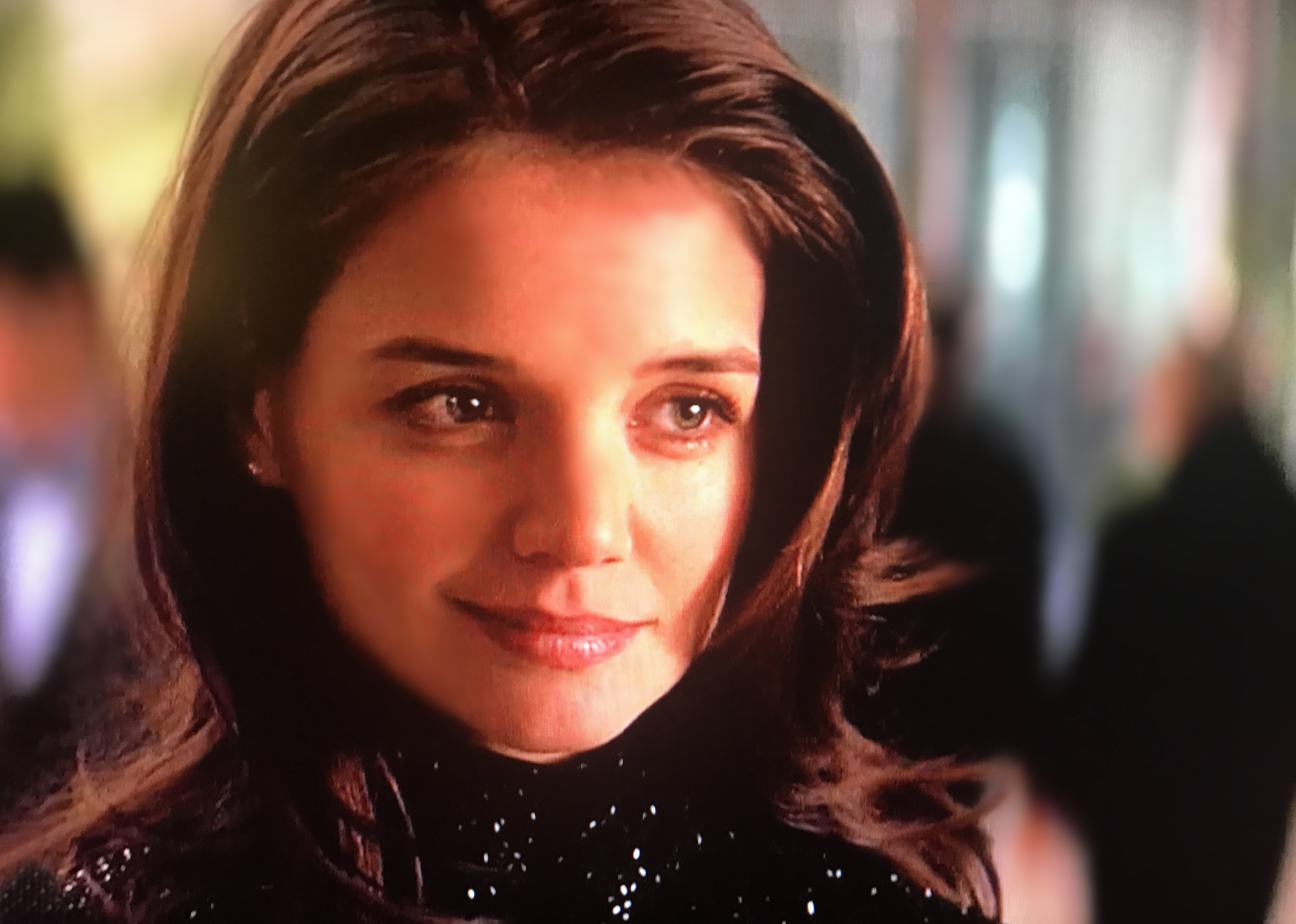The image features a close-up of a young woman, identified as Katie Holmes, who is likely in her 20s. She is positioned towards the middle left of the frame. Katie is wearing a sparkling black dress that extends up to her neck, although only the upper section of her body, from her head to just below her neck, is visible. She has long, wavy brown hair that is parted slightly to the right and cascades down to her shoulders, tapering and waving outward at the ends. Her eyes are open and looking to the right, with a gentle half-smile on her face, but she is not making direct eye contact with the camera.

The background is out of focus, creating a blurred and streaky effect. The upper left-hand corner has a yellow hue, while the lower right-hand corner fades to black. White and blue streaks, as well as red and green streaks, can be seen around her, contributing to the abstract backdrop. Additionally, there appears to be a shadowy figure in the center background with black hair, wearing a white shirt and a black suit jacket. On the right-hand side of the background, two very blurry individuals are visible, also dressed in dark suits, seemingly moving away from the main subject. The overall effect is one of contrast between the detailed image of Katie Holmes and the indistinct, colorful backdrop.